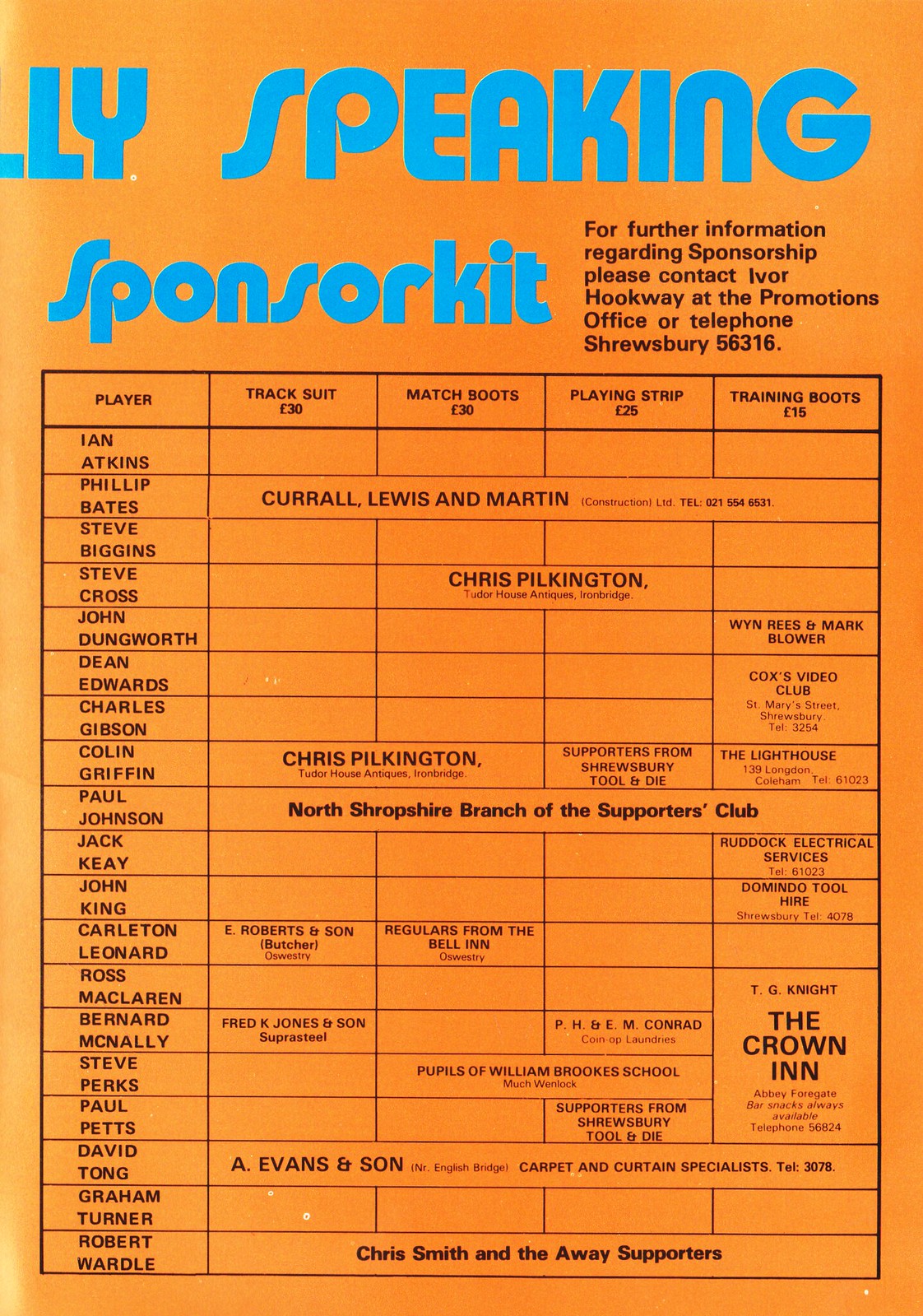This image depicts the second page of a sponsorship program or card with an all-orange background and distinctive bright blue and black text. The top half of the page features a partially cut-off title reading "L-Y Speaking" followed by "Sponsor Kit." Beneath this, there's a detailed contact line in black text stating, "For further information regarding sponsorship, please contact Ivor Huque at the Promotions Office or telephone at Shrewberry 56316."

Central to the page is a comprehensive grid listing players' names such as Ian Atkins and Phillip Bates along the left column. The grid is organized into several headers for different items like Track Suit, Match Boots, Playing Strip, and Training Boots, each accompanied by their respective sponsorship costs. Many cells in the grid are filled, indicating sponsorship contributions, such as The Crown Inn sponsoring the training boots of players like McMullerland, McNally, Perks, and Pets. Other sponsors include individuals and entities like Chris Pilkington and A. Evans & Son.